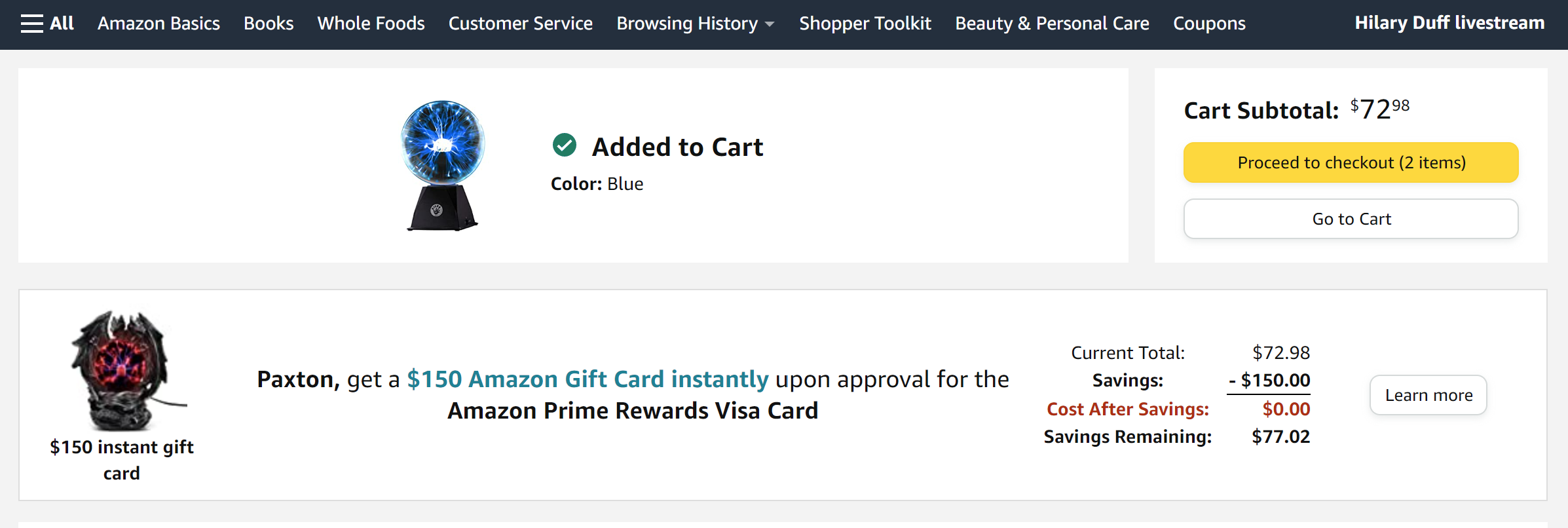An Amazon webpage is displayed, showing confirmation of an item added to the cart. A small green circle with a check mark accompanies the message, "Added to Cart," accentuated in blue. The item appears to be a plasma ball, characterized by static lightning-like patterns when touched.

The familiar black Amazon header stretches across the top, featuring a hamburger menu icon on the upper left. Adjacent categories include "All Amazon," "Books," "Whole Foods," "Customer Service," "Browsing History," "Shopper Toolkit," "Beauty & Personal Care," "Coupons," along with a "Hillary Duff Livestream" on the upper right.

Displayed prominently is the cart subtotal of $72.98 with a yellow button labeled "Proceed to checkout (2 items)" underneath it. Below, the option to "Go to Cart" suggests multiple items are present, although details of the additional item remain unspecified.

The account appears to belong to someone named Paxton. There is an advertisement for the Amazon Prime Rewards Visa Card, offering an instant $150 gift card upon approval. Current total savings and potential future savings are detailed: "Current Total: $72.98," "Savings: -$150," leading to a "Cost after savings: $0," with "Savings remaining: $77.02." A "Learn More" button is placed to the right for additional information on the offer.